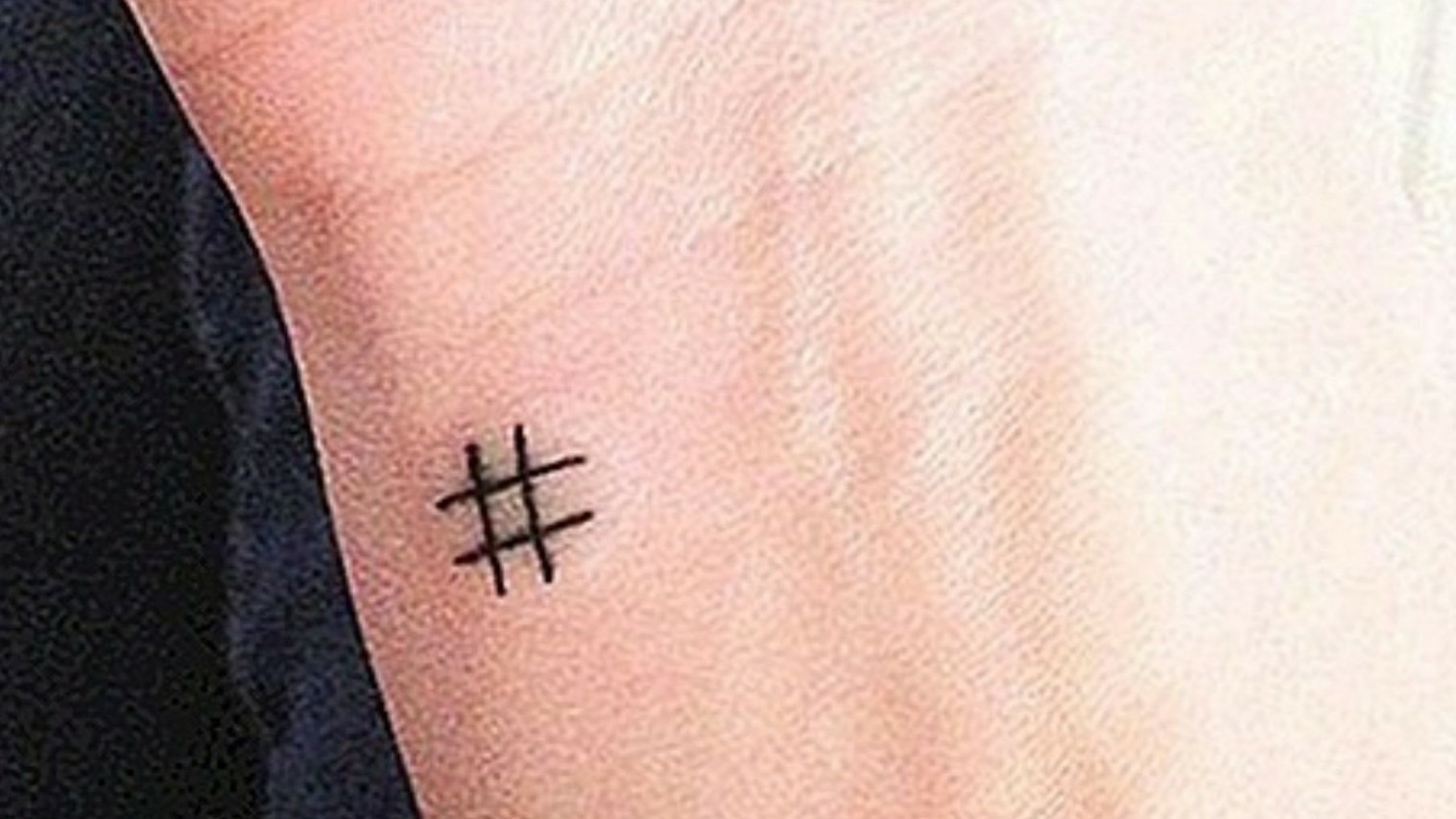This detailed image is an extremely close-up depiction resembling a painting of the inside of a right wrist, turned palm-side up. At the left side of the wrist, there's a simple black tattoo, or possibly a rough burn mark, shaped like a pound sign (#), reminiscent of a tic-tac-toe grid. The design consists of two vertical and two horizontal lines, situated just below where the palm begins. The skin is bumpy and visibly veined, with a prominent bone noticeable in the middle of the wrist. The background is composed of different shades of black, and the arm appears to be resting on a piece of dark cloth.